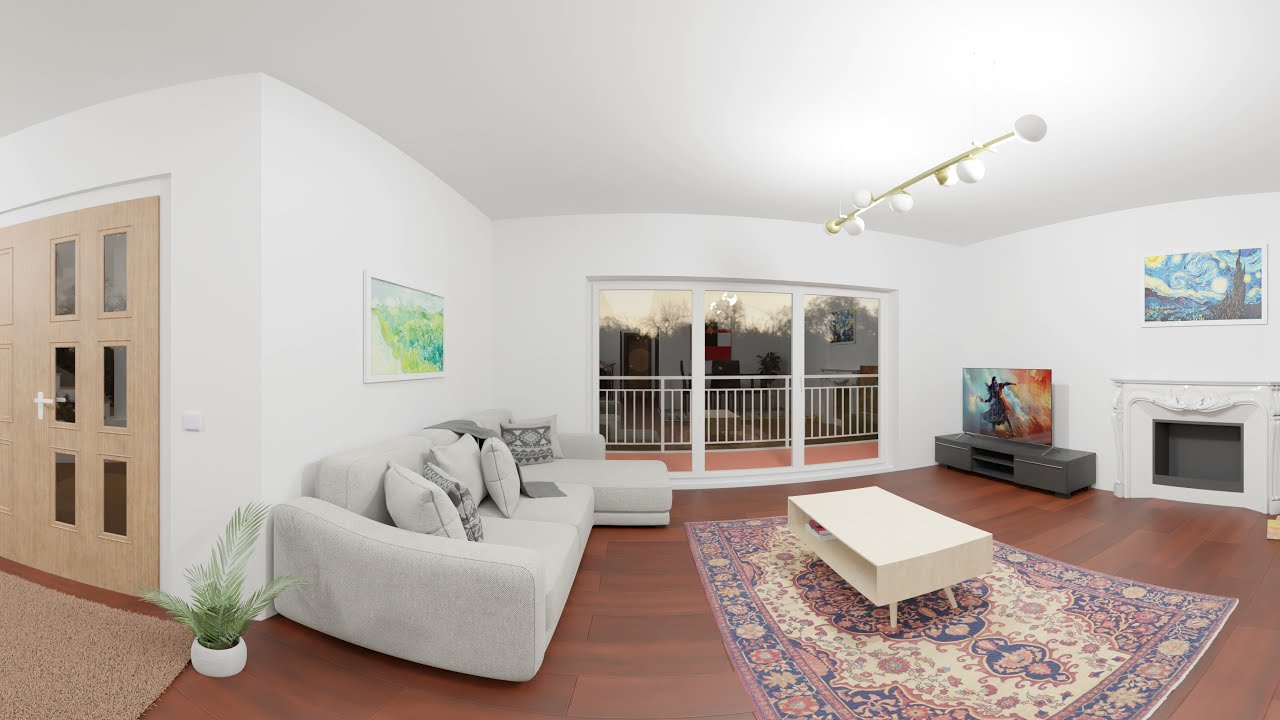This image showcases a sleek, bright white living room with a minimalist design. The space features a square layout with pristine white walls and ceiling, complemented by a rich, dark wood-planked floor. To the left, there are two light pine or beige double doors adorned with six long, narrow glass panes in a grid pattern. In front of these doors lies a small tropical plant in a white planter, its long leaves adding a touch of greenery.

As you move into the living room, you immediately notice an L-shaped light gray couch adorned with white and dark gray cushions, some featuring geometric patterns. The couch offers a chic lounge area. Above it, a rectangular artwork in greens and blues adds a splash of color against the white wall.

Directly across from the couch is a sophisticated entertainment area, complete with a low-profile, sleek gray TV stand and a flat-screen TV displaying a colorful image. A prominent white fireplace with a decorative arch and patterns takes center stage, adorned with Van Gogh's "Starry Night" in yellows and light blues, hanging just above it.

The far side of the room features three large sliding glass doors leading to a balcony with a white railing, allowing ample natural light to flood the room. Underneath the coffee table, a large, ornate rug with cream, blue, and beige hues ties the room together. The coffee table itself is modern, rectangular with angled legs and an open storage space underneath.

This description captures a harmonious blend of pristine white elements, accented by neutral tones and vibrant art, creating a sleek yet cozy atmosphere.